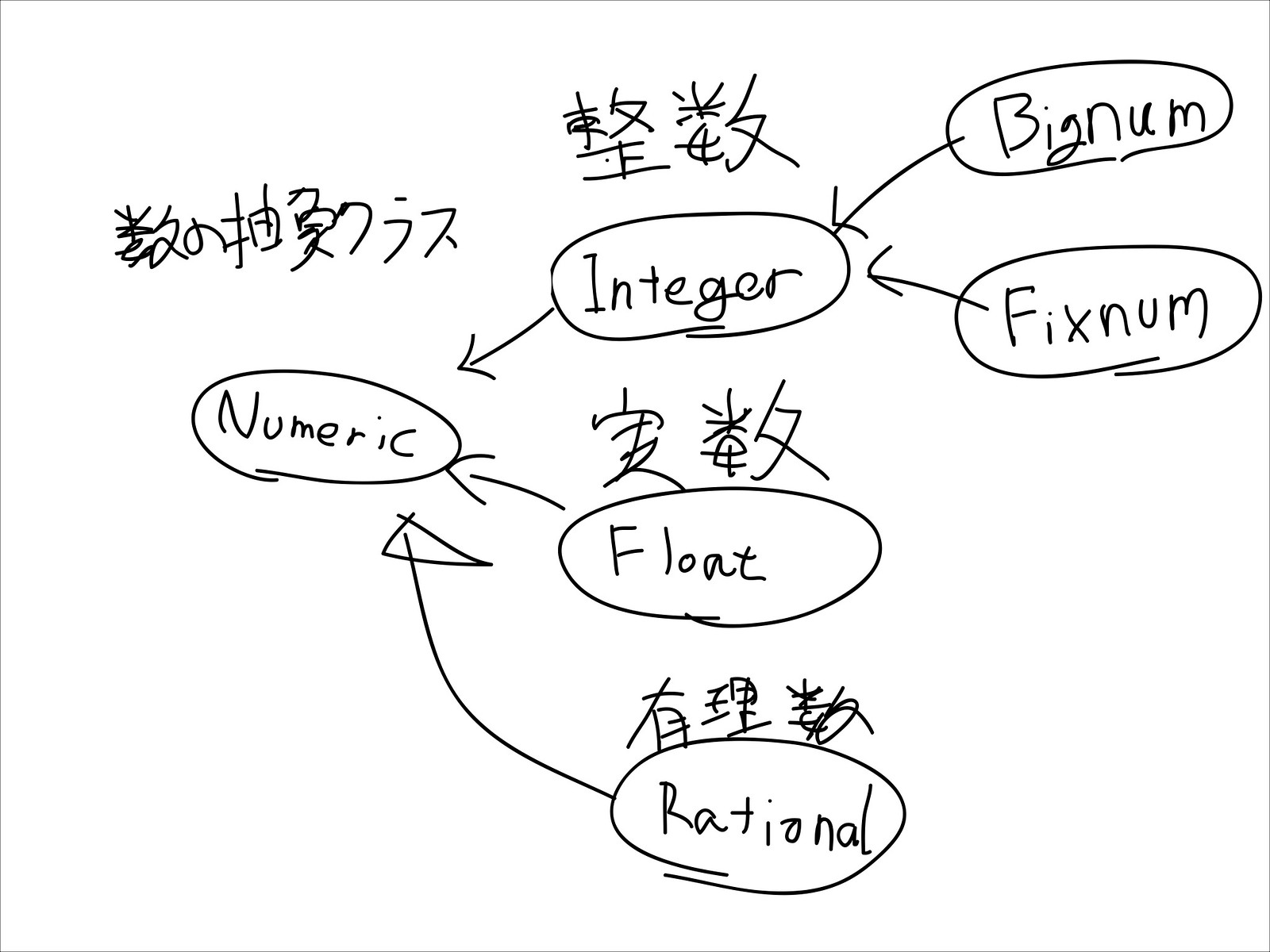The photograph showcases a black-and-white sketch featuring a handwritten mathematical diagram on a pure white background. The diagram, seemingly drawn with a marker, consists of oval-shaped nodes, each containing a word that represents different types of numbers in a programming context. From top to bottom, the English words inscribed within the nodes are: BIGNUM, FIXNUM, INTEGER, FLOAT, and RATIONAL. Each node is connected by arrows pointing to a central node labeled NUMERIC, indicating a hierarchical structure. Notably, there are lines of text in an Asian language above some of the nodes, which likely provide additional context or translations. The diagram prominently displays components such as BIGNUM and FIXNUM at the top, both pointing to INTEGER, which in turn points to NUMERIC. FLOAT and RATIONAL nodes are also connected to NUMERIC. The structure lacks a starting or stopping point and is characterized by the absence of equal signs, suggesting that it serves to identify and categorize types of numerical data rather than solve equations.